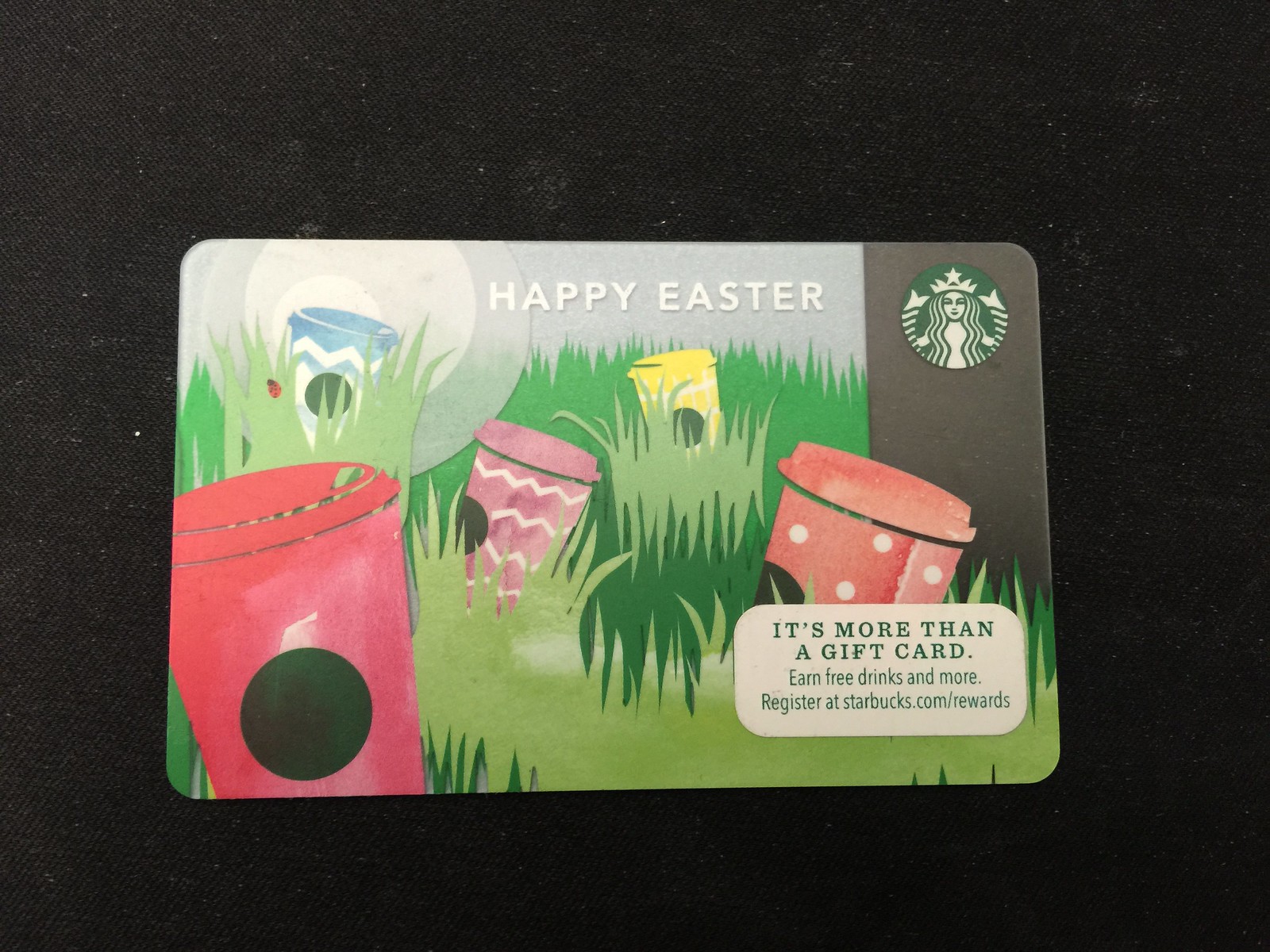This is an image of a festive Starbucks gift card centered against a black background. The card features a grayscale bar vertically aligned on the right side, with the iconic Starbucks logo—depicting the mermaid with long hair, raised arms, and a crown—at the top. Prominently displayed at the top left in white capital letters are the words "Happy Easter." Below this, a cartoon-style grassy field in varying shades of green spans across the card. Nestled within the grass are five colorful coffee cups: a medium blue cup with white zigzags, a bright pink cup, a vibrant yellow cup, a solid red cup, and a pink-red cup adorned with white polka dots. Additionally, a white label is visible at the bottom right corner of the card.